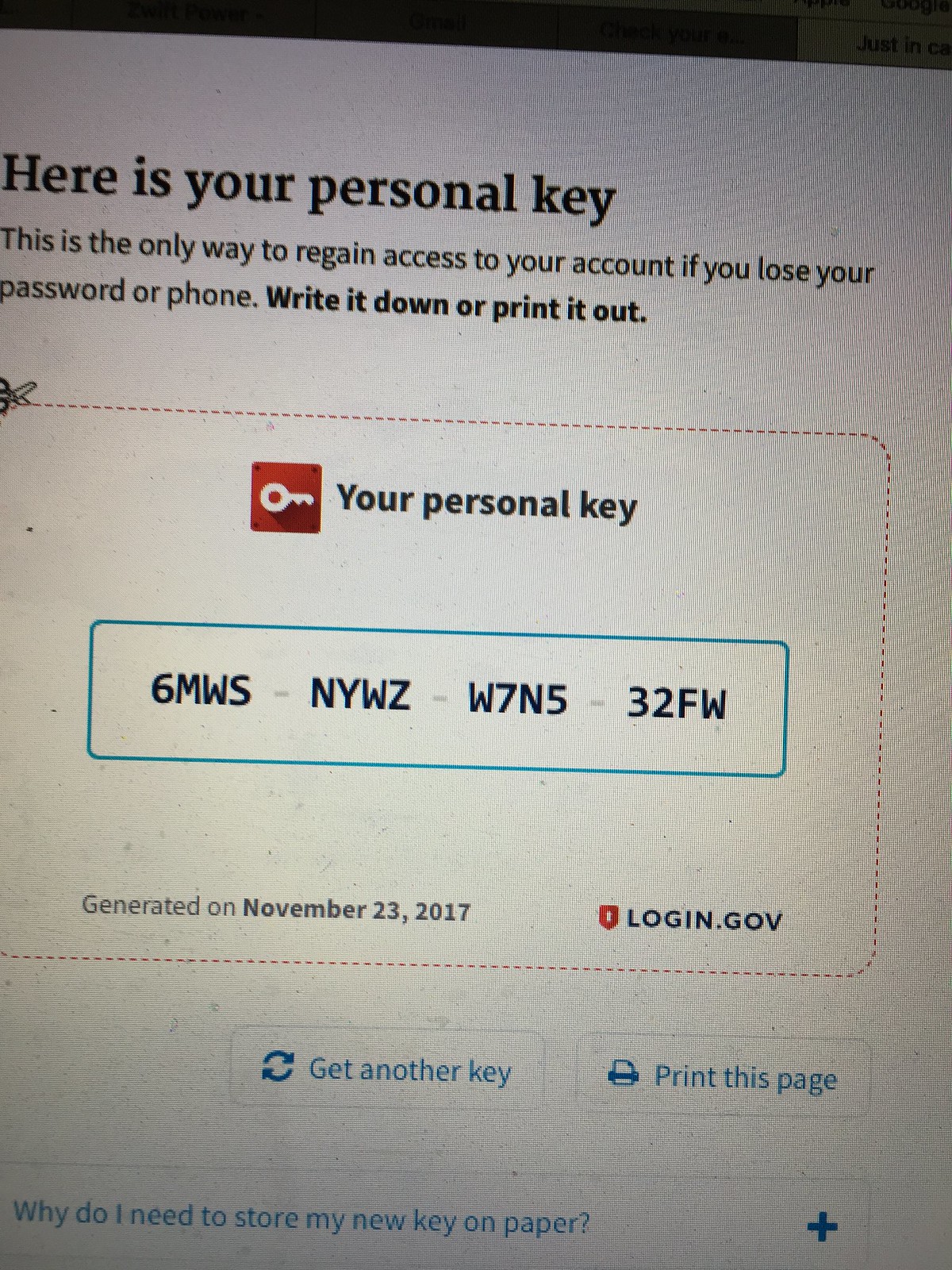The image depicts a photograph of a computer screen, likely showing a security-related webpage from a bank or a service like login.gov. The image has some visible glare and dirt, distinguishing it from a pure screenshot. The webpage features a white background with some noticeable screen glare or striping. Prominently, it displays a message in bold: "Here's your personal key. This is the only way to regain access to your account if you lose your password or phone. Write it down or print it out." Below this message, within a red-bordered area with a cutout design and a key icon, it reads "Your personal key." The personal key is shown in a blue-bordered box and formatted as 6MWS-NYWZ-W7N5-32FW, which was generated on November 3rd, 2017. Other notable elements include a login.gov logo and options at the bottom of the page in light blue: "Get another key" and "Print this page." Additionally, there is a question prompting the user, "Why do I need to store this new key on paper?"